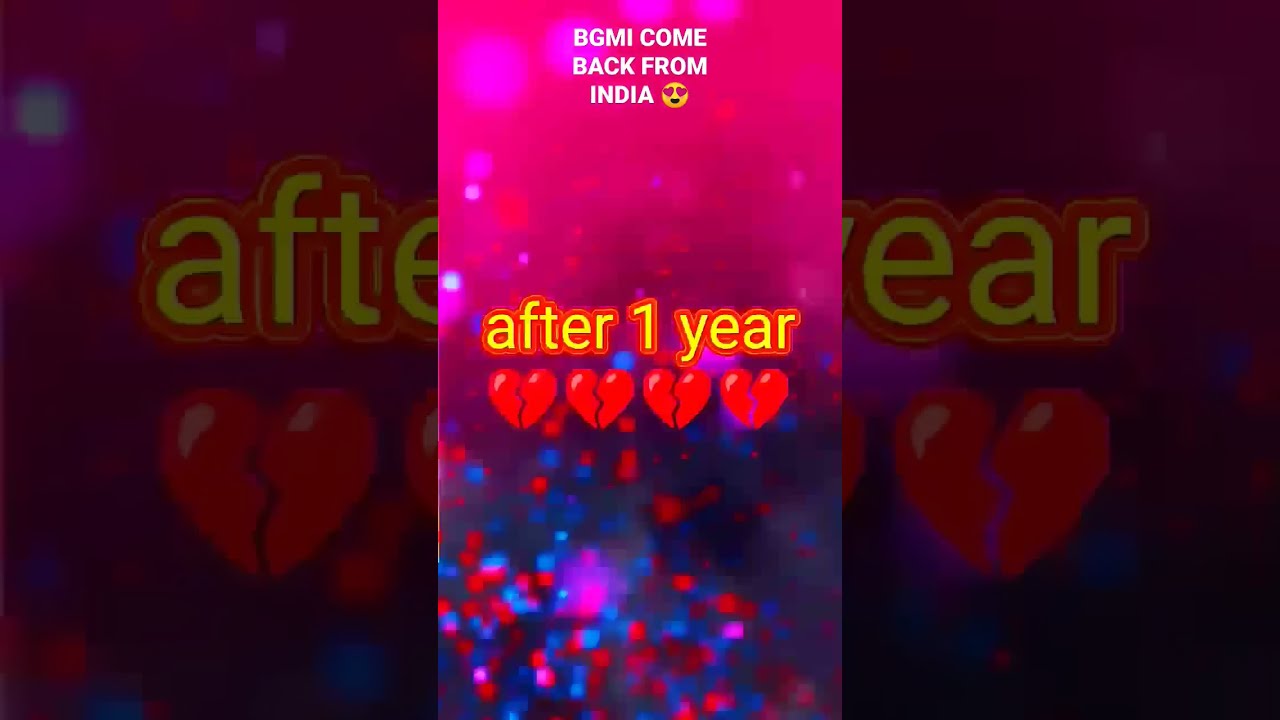The image is a visually striking, computer-generated social media post that employs a layered, double-exposure technique. The main background features a pink-to-blue gradient adorned with sparkles and stardust at the bottom, accompanied by a palette of red, pink, blue, and dark blue hues. Overlaid on this backdrop is a smaller, brighter, and bolder version of the same image, which focuses on specific textual elements.

At the very top of the image, in white bold lettering, it says "BGMI come back from India," followed by an emoji with heart eyes. Below this, in the middle section, the words "after one year" appear in a yellow font, with four red broken hearts aligned beneath it. The smaller overlay obscures part of this text, revealing only "AFTE" and "EA ar," along with partial views of two of the broken hearts.

The background image appears darker and less in focus, creating a shadow effect around the brighter, smaller overlay, which houses the core message of the post. The meticulous design elements, such as the gradient, sparkles, and varying colors, intricately frame the textual content, enhancing the emotional weight of the message through the repeated motif of broken hearts and the return announcement.